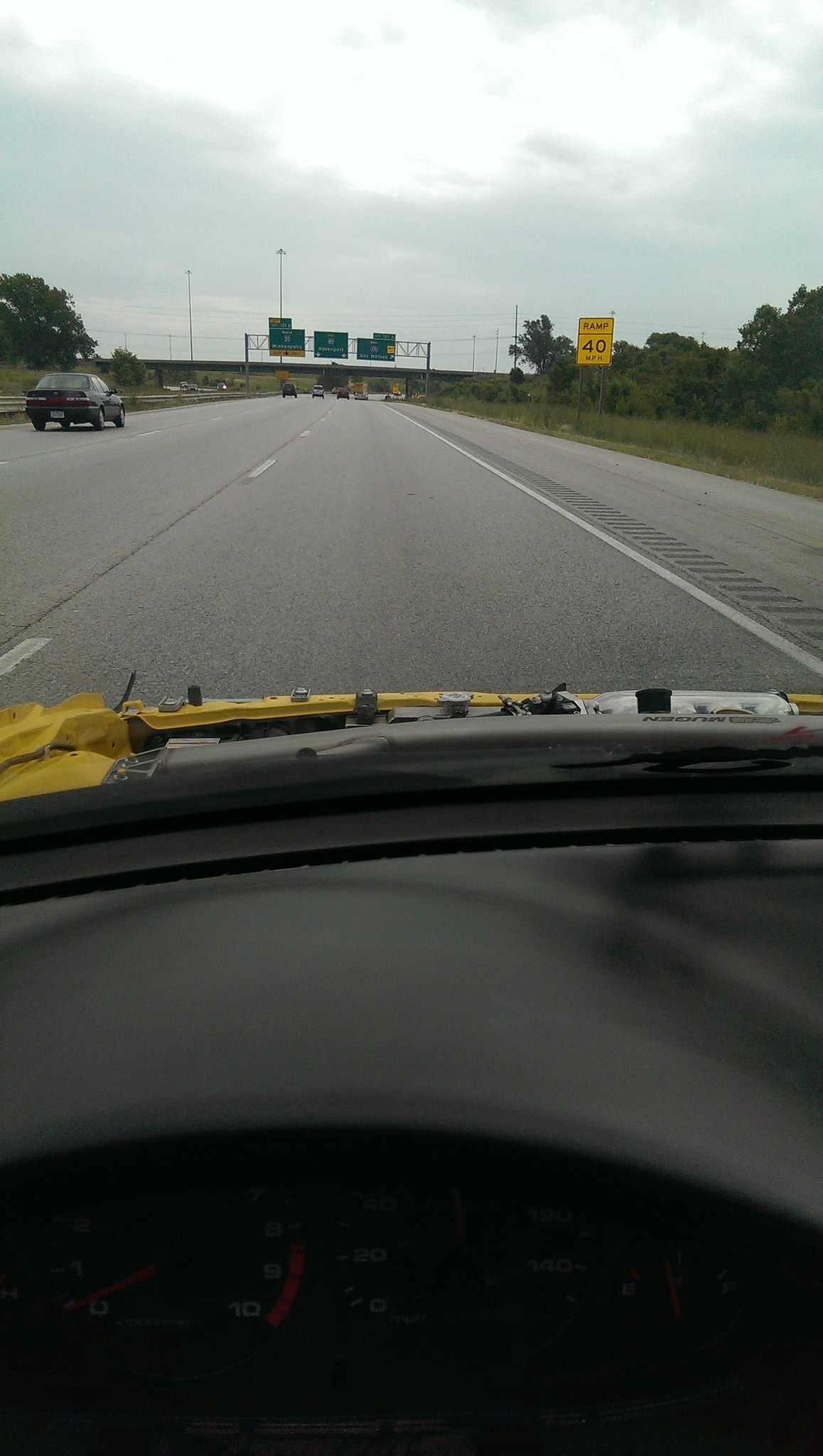A photo captures the interior of a vehicle, showcasing a plastic dashboard with visible gray or black windshield wipers. Through the windshield, a bright yellow car hood is prominently seen. The road ahead is paved in gray, marked with white dashed lines, and has a solid white line on the right side. Adjacent to the road on the right is a dry grass area, flanked by a line of trees stretching into the distance. A yellow road sign is visible, indicating "RAMP" at the top and "40 MPH" at the bottom. On the far left, a tree stands beside the road. In the distant background, green highway signs provide directions and information for navigating the freeway and exit routes. The car is shown in motion, driving forward along this road.